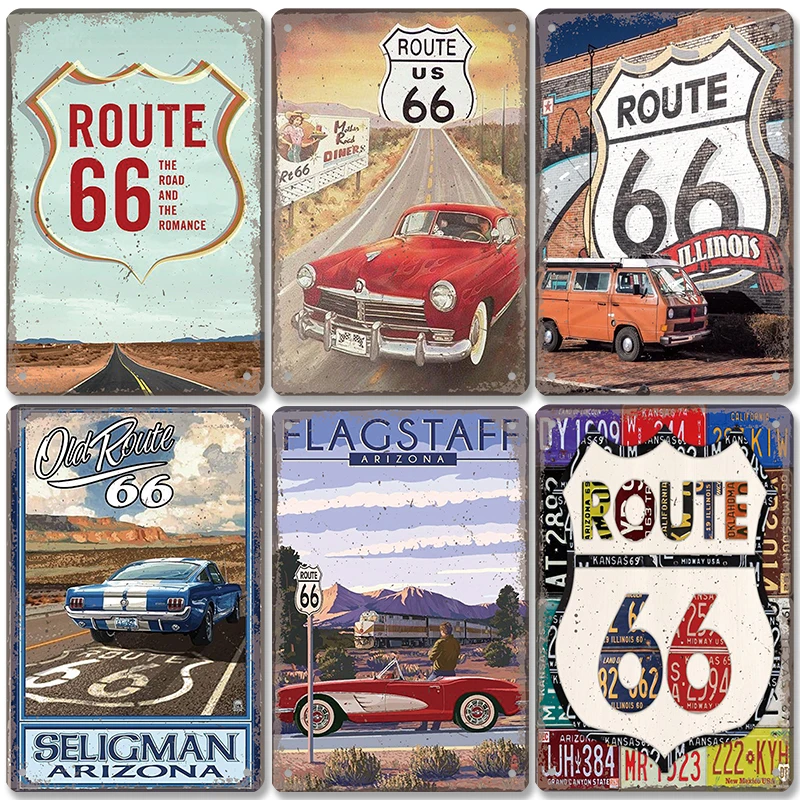The image showcases a collection of six distinct and colorful signs, each celebrating the iconic Route 66, displayed in a grid of two rows and three columns. All signs feature variations of the classic Route 66 shield motif and depict scenes from the legendary highway.

In the top left, a simple, yet evocative design presents the Route 66 marker against a serene blue sky, with an open road stretching into the horizon, framed by dirt paths. The sign prominently reads "Route 66: The Road, The Romance."

To the top middle, a striking black and white Route 66 sign is seen above a red convertible cruising down the highway, emphasizing the spirit of adventure.

In the top right, an old-fashioned orange VW van stands out next to a mural that proclaims "Route 66 Illinois" in a red banner with white text, adding a touch of nostalgia.

The bottom left sign features "Old Route 66" with the iconic logo painted on the road itself, capturing a blue and white car against the backdrop of Seligman, Arizona, evoking a classic desert highway feel.

The bottom middle showcases Flagstaff, Arizona with a red and white convertible Thunderbird against a scenic mountain backdrop, highlighting the classic Route 66 sign.

Finally, the bottom right sign is a creative collage featuring the Route 66 shield overlaid on various colorful license plates, celebrating the diverse journeys along this historic route.

Each of these art deco pieces captures different elements of the Route 66 experience, from bustling road adventures to tranquil desert vistas, making them perfect decorations for any travel enthusiast's wall.